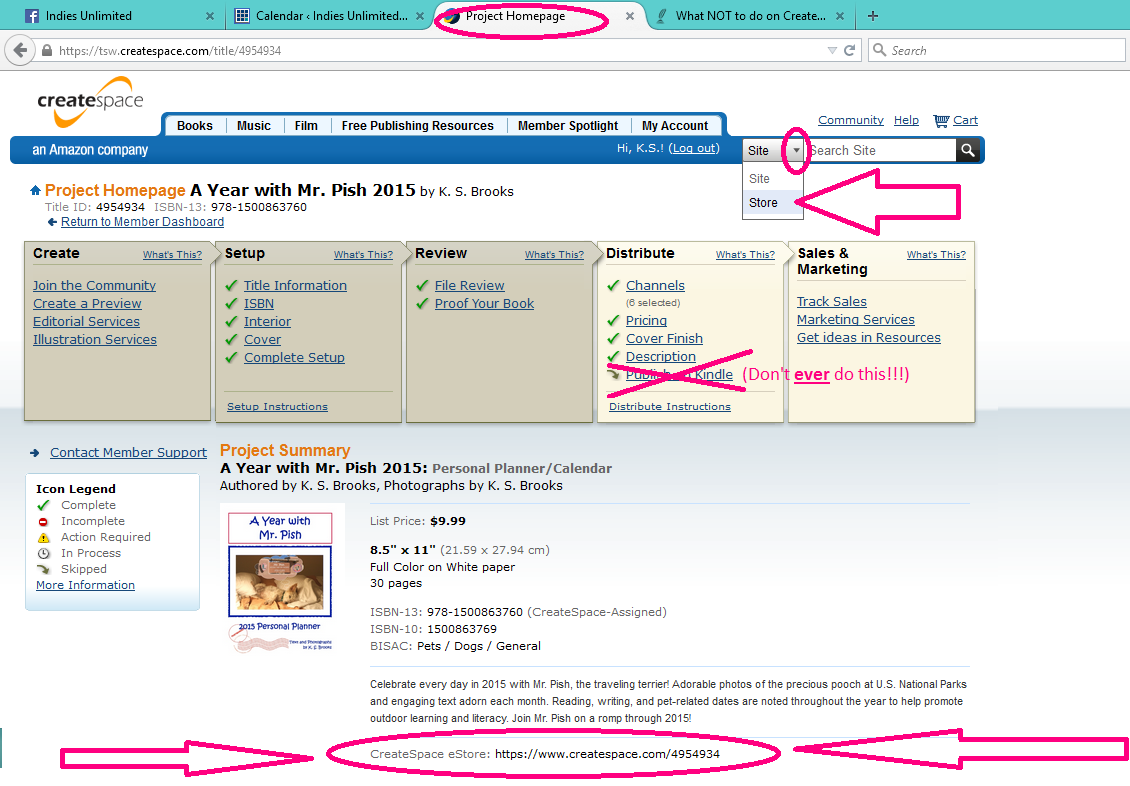This is a detailed screenshot of a web browser with four tabs open. The currently active tab is highlighted with a red circle, titled "Project Homepage."

1. **Tabs:**
   - The first tab shows a Facebook page named "Indeed.Unlimited."
   - The second tab is a calendar also labeled "Indeed.Unlimited."
   - The third tab, titled "What Not to Do on Create," is the immediate next to the highlighted tab.
   - The currently active tab (highlighted), "Project Homepage," is displayed.

2. **Content of the Active Tab (Project Homepage):**
   - The top left corner features the Create Space logo, adorned with yellow squashes.
   - Adjacent to the logo is a navigation bar with links to "Books," "Music," "Files," "Free Production Resources," "Blue Spotlight," and "My Account."
   - Below this navigation, white text on a blue-black background reads "Amazon Company."
   - On the right side, there is a drop-down menu labeled "Site and Store," with the "Store" option highlighted and circled in red, accompanied by a red arrow pointing to it.

3. **Main Page Content:**
   -The page title, situated above the main body, is "Project Homepage," followed by the subtitle "A Year Worth List of Fish," credited to "2015 by KS Box." Additional text reads "10-0-RD, Return to Member Dashboard."
   - Below this, there are several labeled boxes: "Create," "Setup," "Review," "Distribute," and "Sales and Marketing."
   - The "Distribute" section is marked with a large red X, and next to this X are the words "Don't Ever Do This."

4. **Footer:**
   - At the bottom of the page, there is a reference to a "Create Space Store," including a link to Create Space.
   - This section is highlighted with a red circle, with two arrows pointing towards it from each side.

Overall, the screenshot details different tabs relevant to the user’s project and provides a pointed warning not to proceed with a specific action in the "Distribute" section.